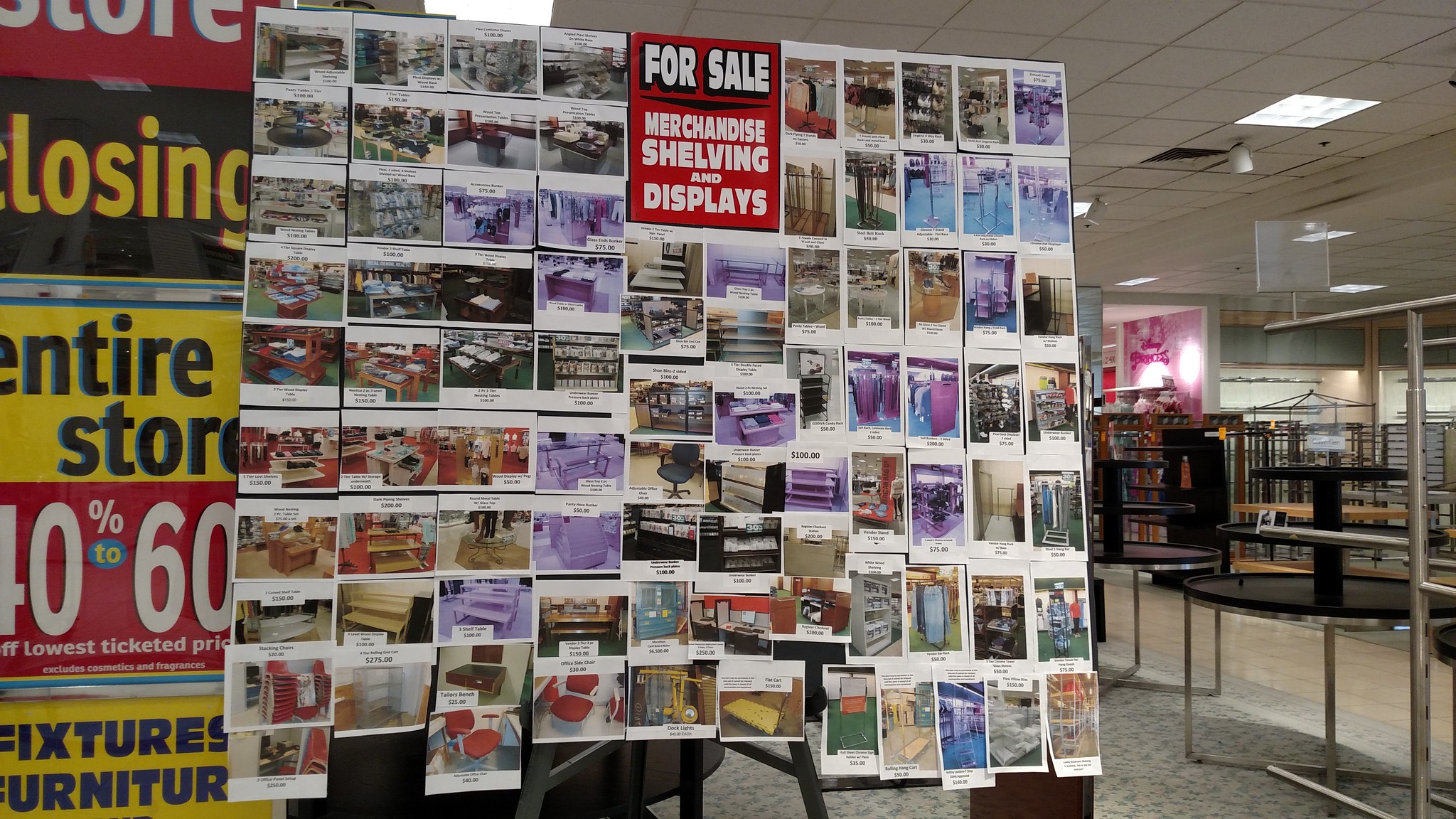This photograph captures a store in the midst of liquidation, evident from the numerous signs proclaiming "Store Closing" and "40 to 60% off." Dominating the scene is a large advertisement sign in the center that reads "For Sale: Merchandise, Shelving, and Displays" in bold red. Beneath this sign, an easel supports a poster board meticulously arranged into a grid-like collage of approximately 110 photos, featuring various store fixtures such as shelves, racks, and even chairs that are also for sale. These photos, arranged roughly 10 high by 11 wide, are colorful and diverse, including reds, purples, and blues with accompanying text details. The surrounding store environment looks quite barren, with mostly empty beige and white shelves and some noticeable gaps where signs should have been displayed. On the left, there is a visible yellow and red sign promoting the clearance, and on the right, parts of the store's white ceiling, lights, and black shelving are noticeable, emphasizing the store's deserted state.